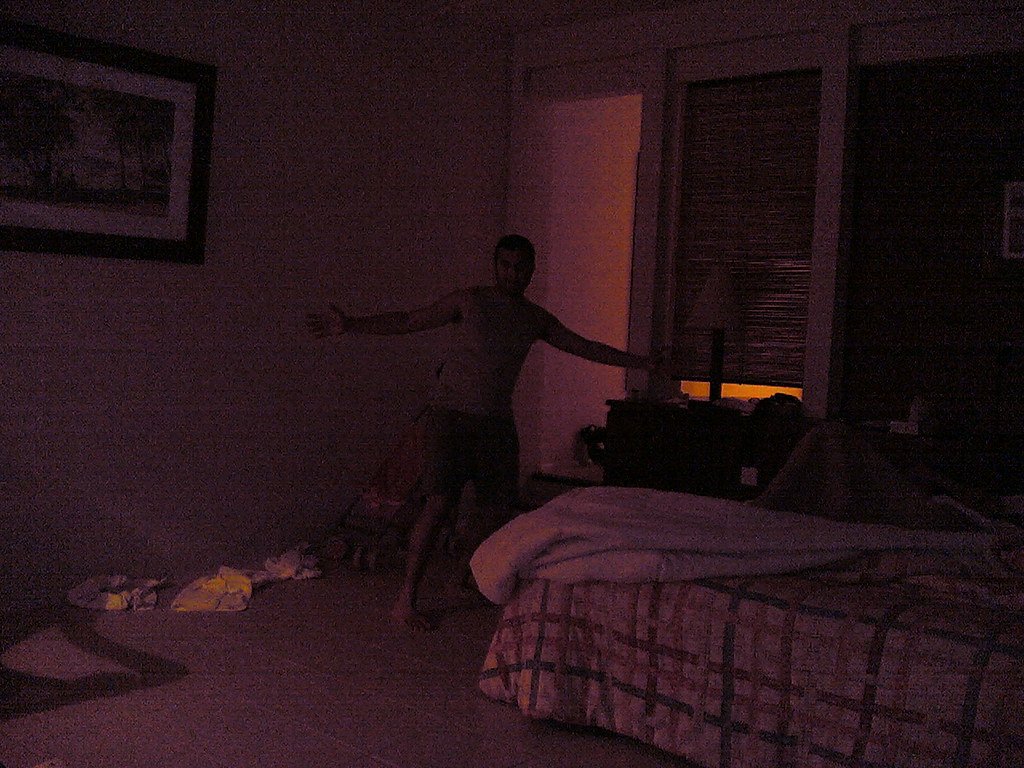In this nighttime bedroom scene, a shirtless man stands centrally, poised with his hands out wide. He is clad in gray shorts and his hair, seemingly brunette, is difficult to discern clearly due to the dim lighting. The room exudes an ethereal glow, bathing everything in a purplish-pink hue. Behind the man, a wall-mounted picture in a black frame, possibly depicting palm trees, adds a hint of decor. The floor beneath him is strewn with dirty clothes, contributing to a casual, lived-in atmosphere. To his side is an unmade bed, its bedspread showcasing an eclectic pattern of black, brown, and pink crosses on a white background.